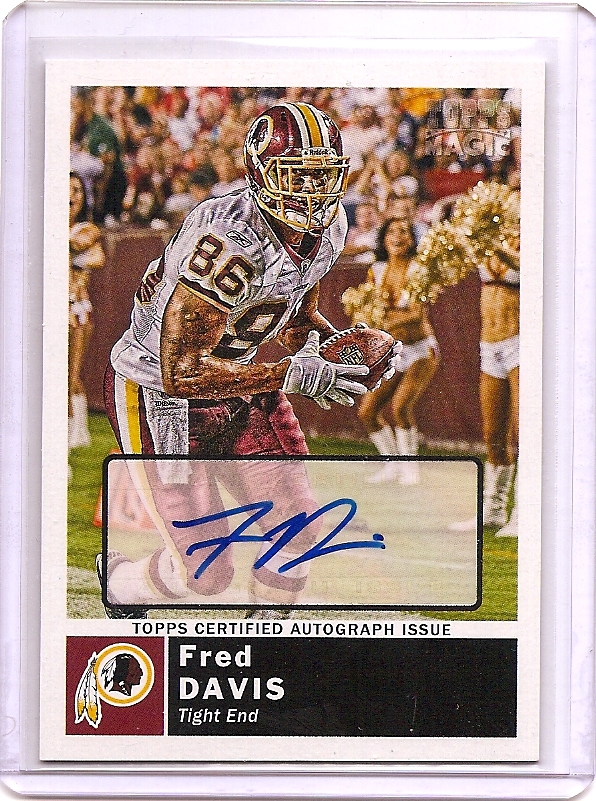This detailed football trading card, preserved in a clear acrylic plastic protective case, showcases Fred Davis, a tight end for the Washington team. The card is framed by the clear case, with a white border lining its edges. A black rectangle at the bottom displays "Fred Davis, Tight End" in white font, flanked by the team's logo: a red square with a white circle bordered in yellow, depicting a profile of a man with two feathers in his hair.

Above this text, in the white border, the card reads "Top Certified Autograph Issue" in black text. The card features a photograph of Fred Davis in mid-run, clad in a white uniform with the number 86, and red, yellow, and white pants, holding a football. There are cheerleaders in white outfits with boots visible in the background. Fred Davis' autograph, an "F" and "D" in blue marker, is prominent in a semi-transparent, white box above the text. Despite minor scratches and flaws, the card remains in good condition, exuding a vintage charm.